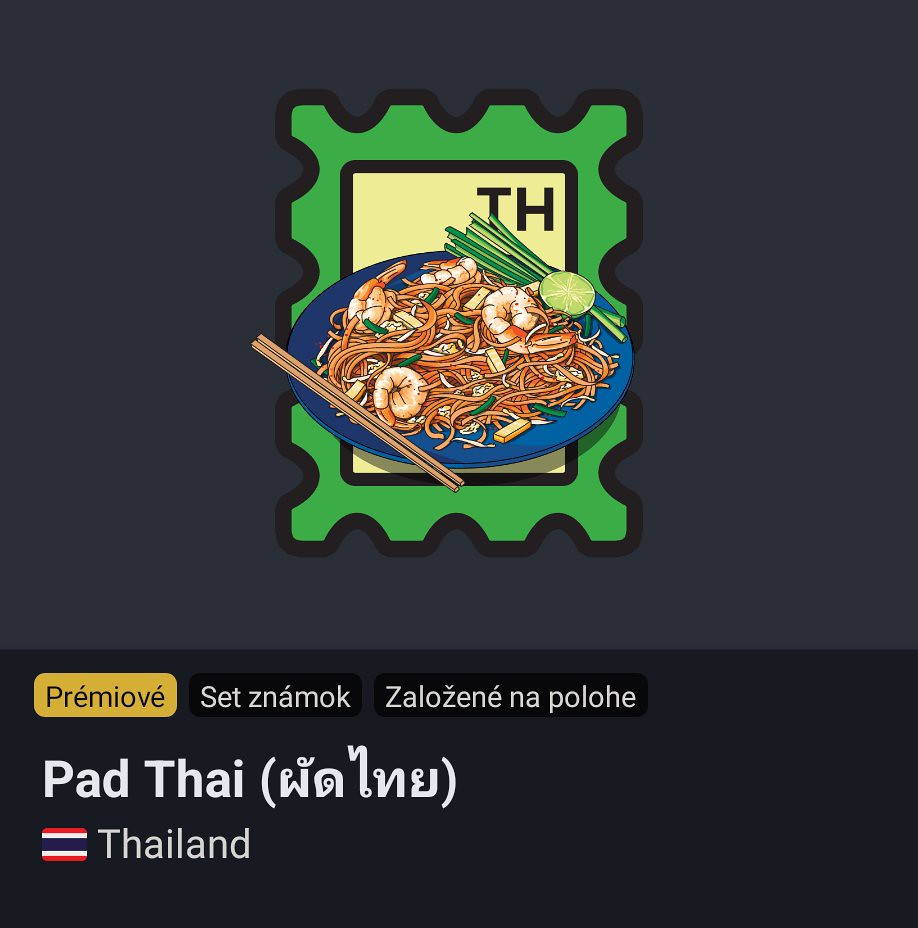This square image presents a detailed, animated graphic that is likely a preview for a registrant from an ad or an app. Central to the colorful design is a large, green postage stamp with a notched border. Within the stamp is a pale yellow rectangle, bearing the letters "TH" in the top-right corner. In front of the stamp, a vivid blue plate holds an appetizing depiction of a shrimp stir-fry, presumably Pad Thai, complete with noodles. The plate also features a pair of chopsticks on the bottom left. To the right of the plate, towards the top, are ingredients including green onions (or leeks) and a lime, adding to the culinary theme. The bottom part of the image includes a series of text boxes resembling tags, one of which is highlighted in yellow with the word "PRIMOVE". Below this, in black text, it says "Pad Thai", followed by "Thailand" and an adjacent Thai flag, consolidating the image's connection to Thai cuisine.